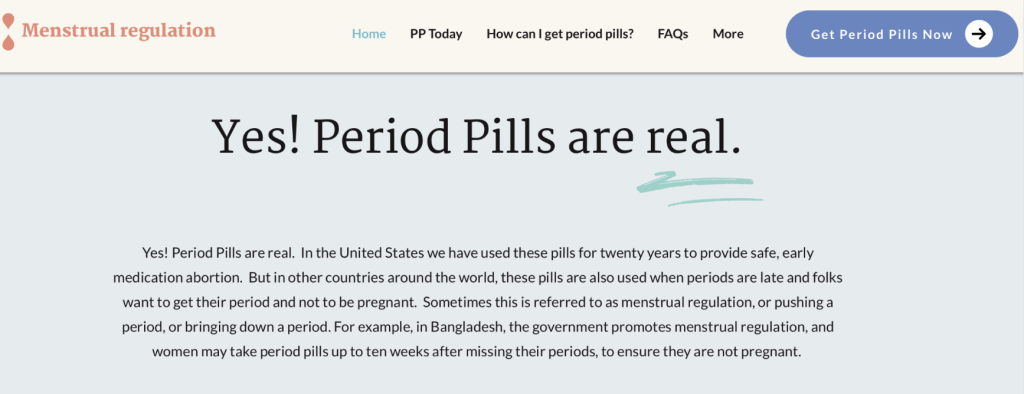This image is a cropped screenshot of a website dedicated to menstrual regulation. The top section features a light pink header with the logo for "Menstrual Regulation" prominently displayed in dark pink on the top left. To the right of the logo, five navigation categories are listed: "Home" (highlighted in blue), "PP Today," "How Can I Get Period Pills," "Facts," and "More." On the far right of the header is a blue banner button labeled "Get Period Pills Now," adorned with a white circle and a black arrow icon.

The body of the webpage has a blue background. Centered at the top in large black letters is the bold statement: "Yes, Period Pills Are Real." Below this heading is a paragraph of text. Both the left and right edges of the screenshot show partially visible sections of the webpage, while the bottom part has been completely cropped out.